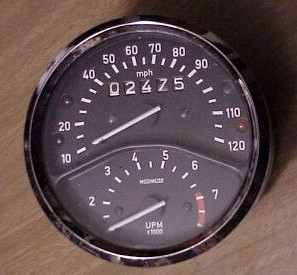This photograph features a compact, circular speedometer set against a dark brown wooden background, which could either be a table or a floor, accented with visible white and dark grains. The speedometer is encased in a black frame with a silver lining at its edge, lending a sleek and classic appearance. Within the speedometer, a black background contrasts vividly with white numerals and letters, interspersed with hints of red for emphasis.

The speedometer's interface is split into two primary sections. The larger, upper section, taking up approximately 60% of the display, marks speeds from 10 to 120 miles per hour. This section is defined by a prominent black border and is equipped with a white needle that points to the speed readings. The lower, smaller section is designated for the tachometer, marked with "UPM x1000." This section starts presumably at 1 (though the number 1 is missing) and spans from 2 to 7, indicating the engine's RPM. As the readings approach 7, the background transitions to red, signaling the higher, more critical engine speeds.

Despite the image's small size and some details being hard to discern, the speedometer's design and the intricate details of both the speed and RPM sections are noticeably clear.